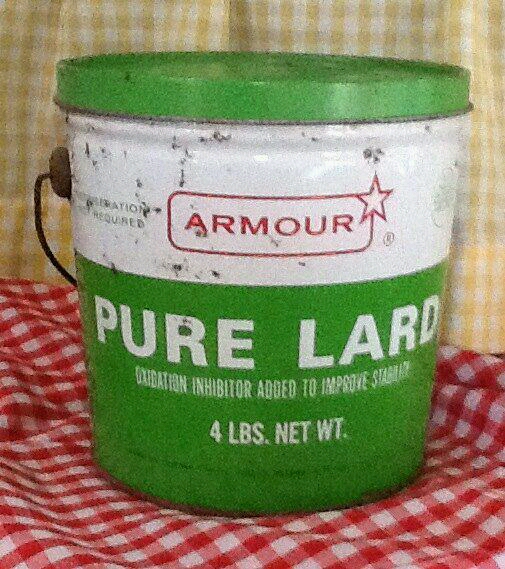This detailed photograph showcases a tub of lard prominently positioned on a red and white checkered cloth. The tub features a vivid green lid, seamlessly complemented by a wide white band below it. On this band, an eye-catching logo reads "Armour" in bold, red font accompanied by a five-pointed star on the upper right corner – refining the brand's distinct identity.

To the left of the logo, though partly obscured by small bits of dirt on the tub's surface, appears a notice in black text stating, "Refrigeration is not required." Directly beneath the logo, printed in the same vibrant green as the lid, the text clearly indicates "Pure Lard" in white font, along with the added detail "Oxidation inhibitor added to improve stability." Completing the informative labels, it notes the net weight of the contents as "Four pounds."

The image effectively captures the essence of this classic kitchen staple, juxtaposed against the nostalgic backdrop of the red and white checked cloth.